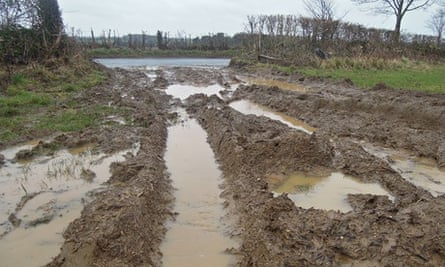The image depicts a photorealistic scene of a rural area following a heavy rainfall. The foreground features a dirt driveway marred by large, muddy furrows created by vehicles. These deep ruts have filled with muddy water, forming a series of puddles stretching toward a body of water in the background, which appears to be either a river or a pond. Surrounding the water, we see a mix of brown, muddy grass and patches of green, but it's clear from the overall lack of foliage and the gray sky that this scene takes place in winter.

Lining the paved road that runs behind the muddy turnoff are uniformly trimmed, leafless hedges or shrubs, indicating it's the winter season. Further in the background, sparse tree trunks and potentially damaged or removed trees can be seen, possibly affected by the recent heavy rains. The entire area is devoid of buildings, vehicles, or people, emphasizing its isolation and the impact of the weather on this desolate landscape.